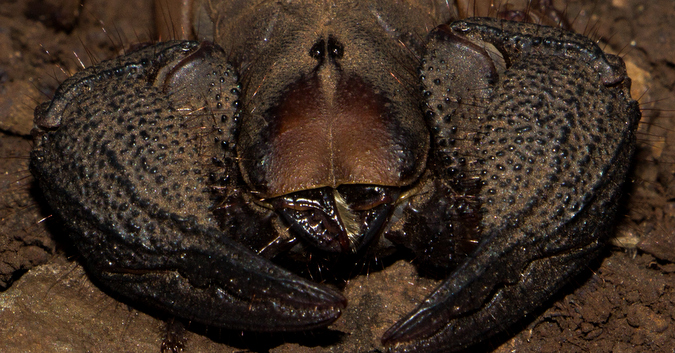This close-up image features a creature that resembles a scorpion or a similar crustacean, potentially even a crab or lobster. The creature is predominantly dark brown and black, its body blending seamlessly with the similarly colored rocky or earthy ground beneath it. Dominating the frame are its two massive claws, each adorned with black bumps and bristly hairs, adding to a somewhat prickly and moist appearance. Between the claws, the mandibles and slimy mouthparts are visible, suggesting an ancient and possibly still or decayed state. Its pair of small, beady eyes are set deep within a hard carapace that transitions from a dark brownish gray to black towards the front. The image is tightly focused on the head and upper body of the creature, with its precise classification remaining ambiguous due to the close-up nature of the photograph.